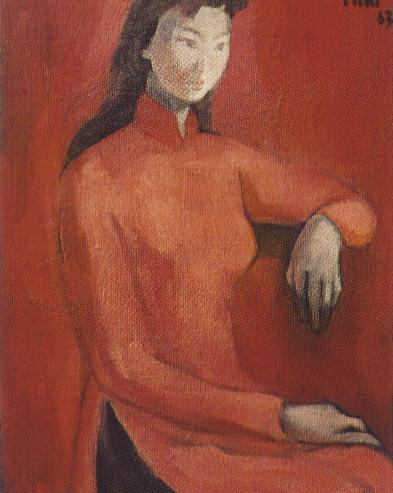This vertical, rectangular painting depicts an almost expressionless Asian woman with pale skin and long, dark brown hair that flows behind her shoulders. She wears an orange, long-sleeved top with a high collar that encircles her neck and forms a small V in the front. The top has a slit at the waist, revealing dark, possibly black or dark gray bottoms. Only her upper body is visible, as she sits sideways in a chair, her left arm resting on the chair's back, and her right hand resting near her lap. The background matches her top, being a slightly darker shade of orange, although some accounts describe it as red. Her serious facial expression is framed by straight bangs and dark eyebrows. Notably, her right breast appears slightly larger than her left. The painting possesses a visible canvas texture, and there's an artist's signature in the top right corner, indicating it may have been created in 1983.